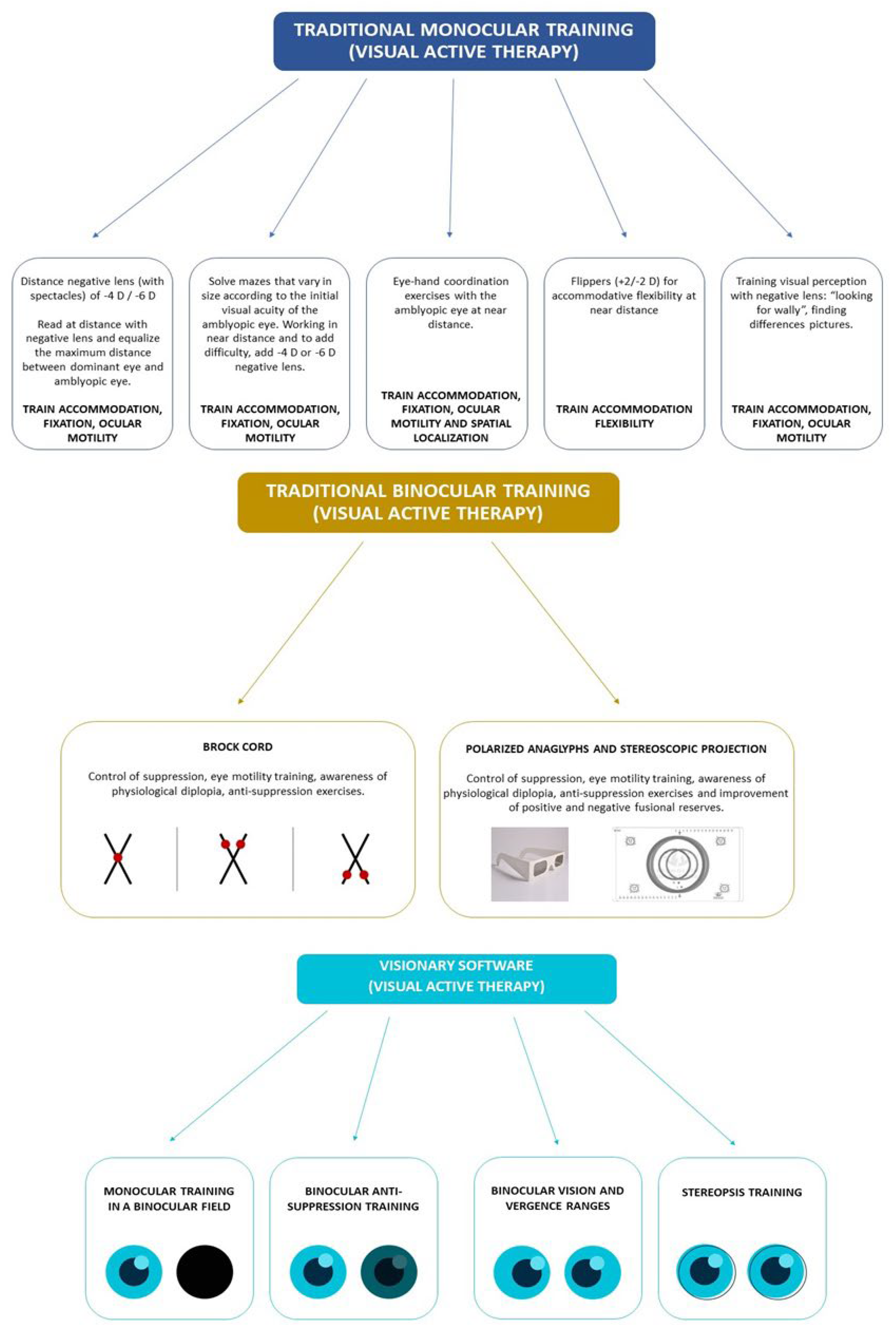The diagram features a comprehensive layout divided into three major sections against a white background, each representing different types of visual active therapy. The first section is marked by a dark blue rectangle with the white text "Traditional Monocular Training" followed by "Visual Active Therapy" in parentheses. From this section, five blue arrows point downward to rounded-corner squares containing detailed information, although the texts are too small to read clearly.

Below this section, a gold rectangle with white text signifies the "Traditional Binocular Training" and is also labeled "Visual Active Therapy" in parentheses. Two arrows extend downward from this section, leading to larger rectangular areas known as "Brock Cord" and "Polarized Anaglyphs and Stereoscopic Projection," each containing images and explanatory text.

The final section at the bottom is a light blue rectangle with the title "Visionary Software" and "Visual Active Therapy" in parentheses. This section features four blue arrows directing to squares below, each indicating different training modules. The first is "Monocular Training in a Binocular Field," with a blue and black circle. The second is "Binocular Anti-Suppression Training" with a light blue and dark blue circle. The third is "Binocular Vision and Vergence Ranges" with two blue circles, and the last is "Stereopsis Training," also illustrated with two blue circles.